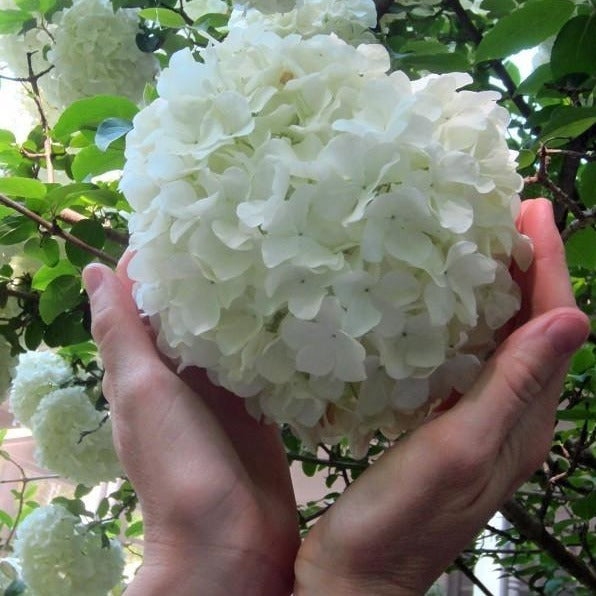In this close-up nature shot, a person is delicately cupping a large, round white flower, known as a snowball bush blossom, in their hands. The flower, resembling a giant puffball or potentially a chrysanthemum, consists of hundreds of tiny petals, creating an elegant and dense appearance. The person’s wrists are together, with their palms open, tenderly holding the blossom. It is a sunny day, as light gently illuminates the flower and the person's hands. Behind the focal bloom, an array of similar white flowers and green branches can be seen, suggesting this plant grows abundantly, likely on a large bush or tree. The background consists of dense green foliage of varying shapes and hues, and there are hints of buildings partially obscured by the branches. The overall scene is brimming with natural beauty and greenery.